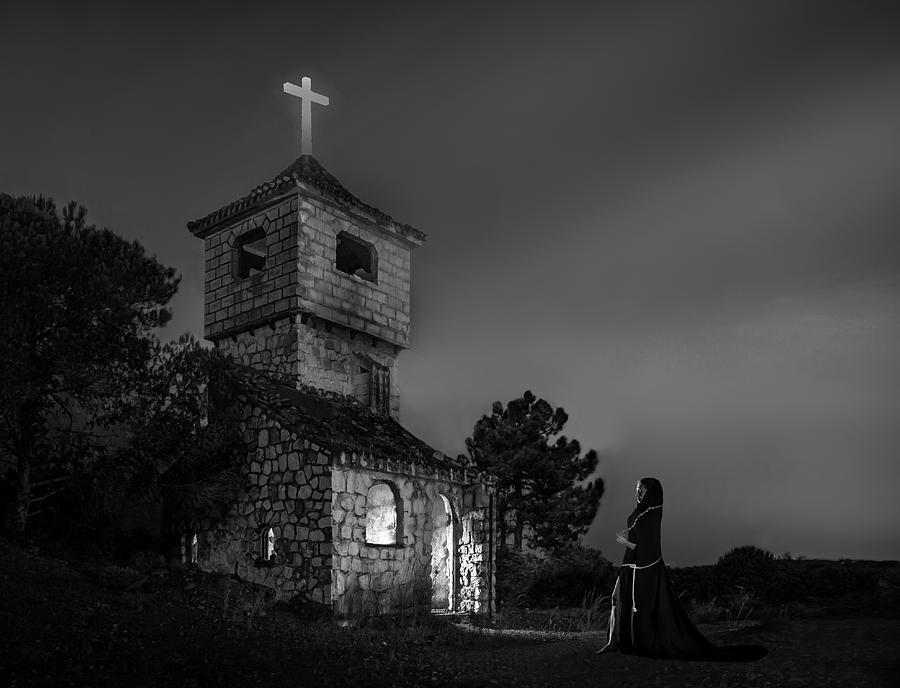This black-and-white photograph captures a small, rustic stone church set against a dark, ominous sky that suggests early 1800s or 1900s. The structure features a distinctive white cross atop a steeple with arched windows on each side. The church has an open arched door and an arched window to its left, both glowing with light from the inside. To the sides and background, dark, shadowy trees frame the scene, adding to the eerie atmosphere.

In the foreground stands a woman, presumably a nun, clad in long black robes and a head covering. She holds a rosary in one hand, with a white rope cinched around her waist. Intriguingly, her bare leg is visible beneath the robe, an unusual touch that contrasts with her otherwise religious appearance. She seems to be either walking towards or standing outside the illuminated church, her figure partially illuminated by the light spilling from the open door. The entire scene evokes a surreal, cinematic quality, reminiscent of a detailed movie set or a hauntingly detailed painting.